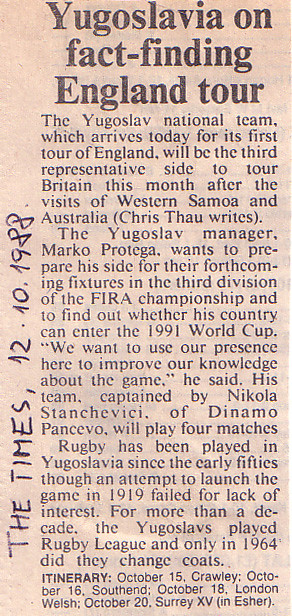The image is an old newspaper clipping with a beige, cream-colored background and black lettering. Dominating the clipping is the headline, "Yugoslavia on Fact-Finding England Tour." This article, authored by Chris Thow, discusses the arrival of the Yugoslav national team for their first England tour, marking them as the third team to visit Britain in the same month, following Western Samoa and Australia. The team's manager, Marko Protega, aims to prepare his squad for upcoming fixtures in the third division of the FIRA Championship and assess the possibility of entering the 1991 World Cup. Protega emphasizes the tour's objective to enhance their understanding of the game. Captained by Nikola Stančeviči of Dynamo Pansevo, the team is set to play four matches. The article also highlights Yugoslavia's rugby history, noting a failed attempt to popularize the game in 1919, a switch to rugby league for more than a decade, and finally adopting rugby union in 1964. The snippet covers the entire image, and on the left side, "The Times 12-10-1988" is handwritten in black pen, indicating the likely date of publication.